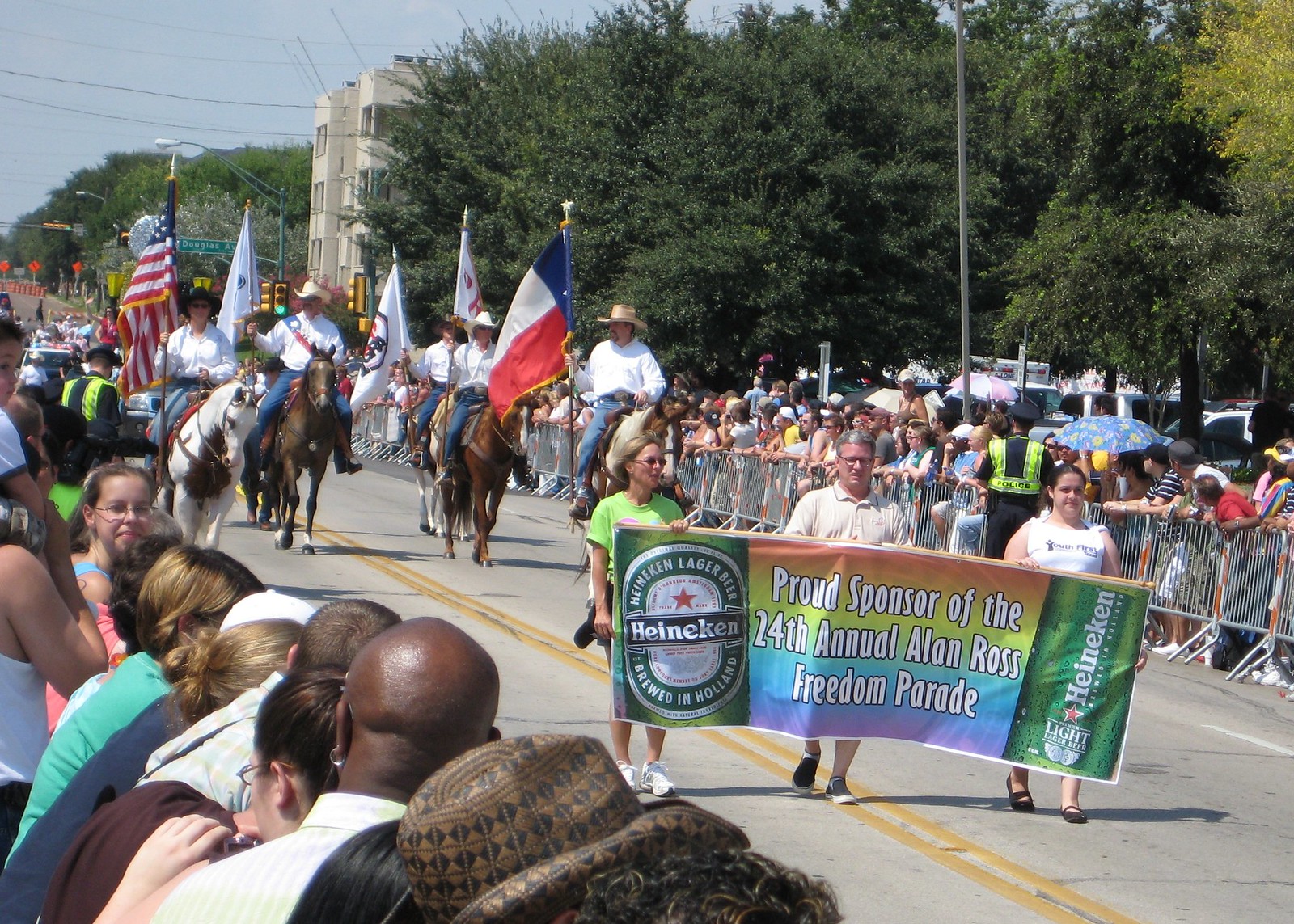This full-color image captures a lively outdoor parade under a sunny sky, likely in Texas, as indicated by one of the flags. Crowds line both sides of the street, watching as participants march down the road marked by a yellow center stripe. Prominently featured in the foreground are three people holding a banner for Heineken, which reads "Proud Sponsor of the 24th Annual Alan Ross Freedom Parade." The banner is flanked by two women on either side and a man in the middle. Just behind them, four horseback riders, adorned with flags, can be seen; the rider on the left carries an American flag while the one on the far right bears the Texas state flag. The vibrant scene, filled with colorful banners and flags, suggests it might be a gay pride parade, celebrating diversity and inclusion.